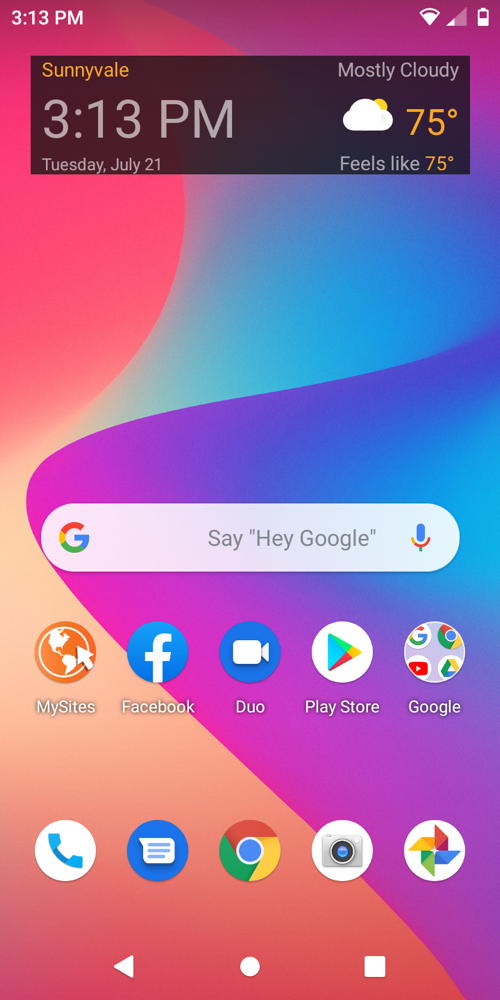This screenshot captures the home screen of an Android phone, providing a detailed view of various elements and widgets.

**Header:**
- **Time:** The top left corner displays the time, 3:13 p.m.
- **Status Icons:** The top right corner features the icons for Wi-Fi, cellular data, and battery status.

**Wallpaper and Notification Bar:**
- The background showcases vibrant swirling patterns in shades of orange, red, blue, and purple.
- The top part of the screen contains a black rectangle displaying essential information:
  - **Location and Time:** "Sunnyvale," "3:13 p.m."
  - **Date:** "Tuesday, July 21"
  - **Weather:** "Mostly cloudy" with an accompanying icon showing a cloud with the sun peeking from the top right.
  - **Temperature:** "75 degrees, feels like 75 degrees."

**Google Search Widget:**
- Positioned centrally on the screen is a rounded rectangle:
  - **Prompt:** "Say 'Hey Google'"
  - **Icons:** The Google symbol on the left and a microphone symbol on the right.

**App Icons:**
- **Top Row (from left to right):**
  1. **My Sites**
  2. **Facebook**
  3. **Duo**
  4. **Play Store**
  5. **Google**

- **Bottom Row (from left to right):**
  1. **Telephone App**
  2. **Messaging App (likely for text messaging)**
  3. **Google Chrome**
  4. **Camera App**
  5. **Google Windmill App** (unspecified application related to Google)

**Navigation Bar:**
- Located at the very bottom of the screen are three standard navigation buttons:
  - **Back Arrow (left)**
  - **Home Circle (center)**
  - **Square App Switcher (right)**

Overall, the screenshot effectively showcases a typical Android home screen layout with time, weather, search functionality, and organized app icons for easy access.